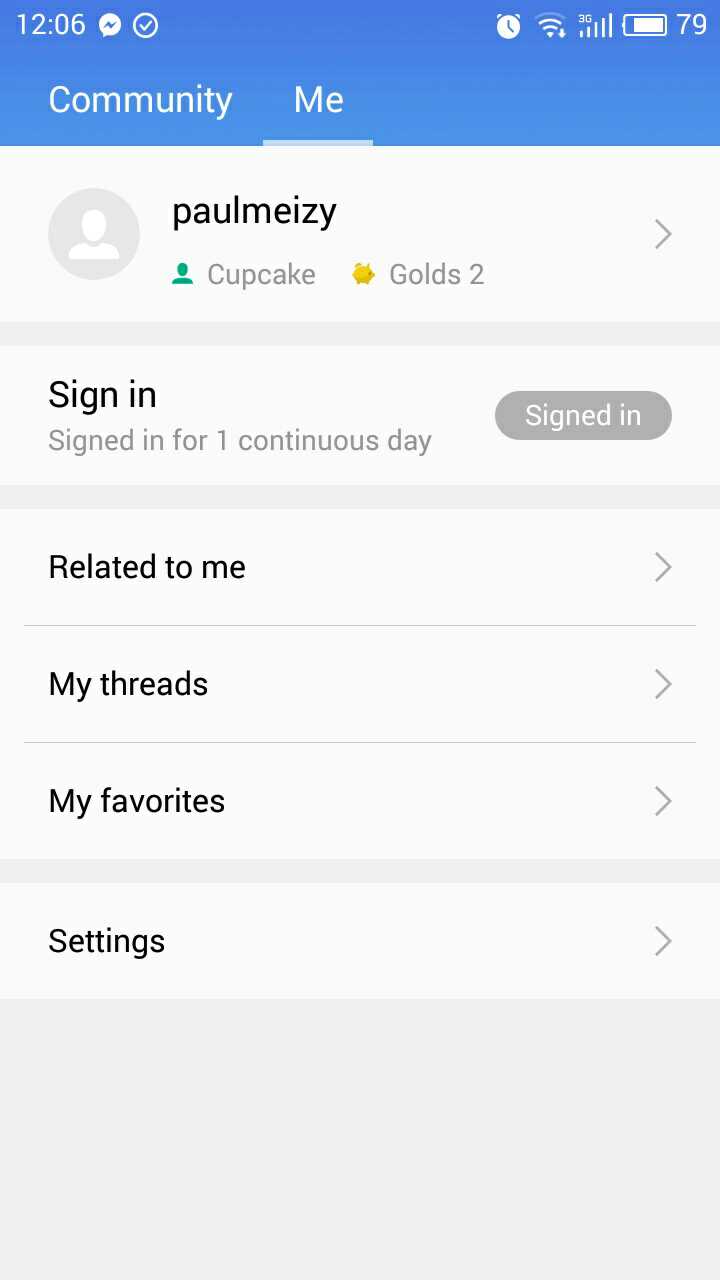This image appears to be a screenshot of a vertically-oriented interface, similar to that of a smartphone.

At the top, within a blue header, the time "12:06" is displayed on the left. Next to the time are icons including a checkmark, a speech bubble with a lightning bolt, an alarm clock, a signal reception icon, a Wi-Fi symbol, a battery symbol indicating 79% charge, and a number '79.'

Beneath the blue header is a white section with the word "Community" in white text, followed by "Me," which is underlined. Below this header, the name "Paul Mazie" is displayed in black text, accompanied by a gray circle containing a white outline of a person on the left.

Further down, there is the word "Cupcake" next to a green silhouette of a person, and to the right, it says "Goals 2" represented by a small gold piggy bank icon. There is a gray arrow pointing to the right next to these elements.

Subsequently, the text reads "Signed in for one continuous day," accompanied by a gray sign-in button. Lower still, the section lists "Related to Me," "My Threads," and "My Favorites," with arrows pointing to the right next to each option. Finally, at the bottom, "Settings" is displayed with an arrow pointing to the right.

The layout and elements seem to structure a user profile or community interface on a mobile device.